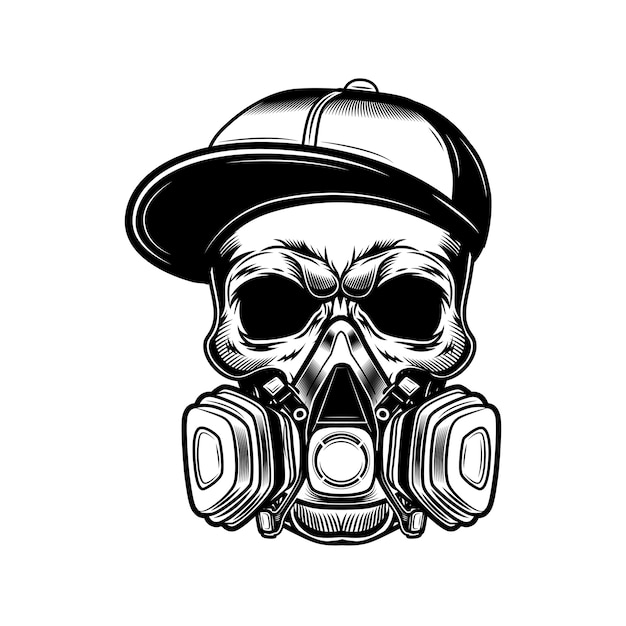Depicted is an intricate, black-and-white digital artwork featuring a menacing skull at its center. The skull's hollow, sunken eyes and furrowed brow convey a scowling, angry demeanor, enhancing its intimidating presence. It dons a sideways-turned baseball cap, with heavy black shading around the edges, particularly on the visor, giving it a solid appearance. Covering the bottom half of the skull’s face is a detailed gas mask with two chambers extending outwards to the left and right. The artwork is meticulously detailed with fine lines and shading, especially around the skull's facial contours and the cap, creating a sense of depth. This piece exudes a grunge, hip-hop aesthetic and could easily serve as a striking logo, tattoo, or sticker design, reminiscent of edgy biker tattoos or iconic band logos like Guns N' Roses.